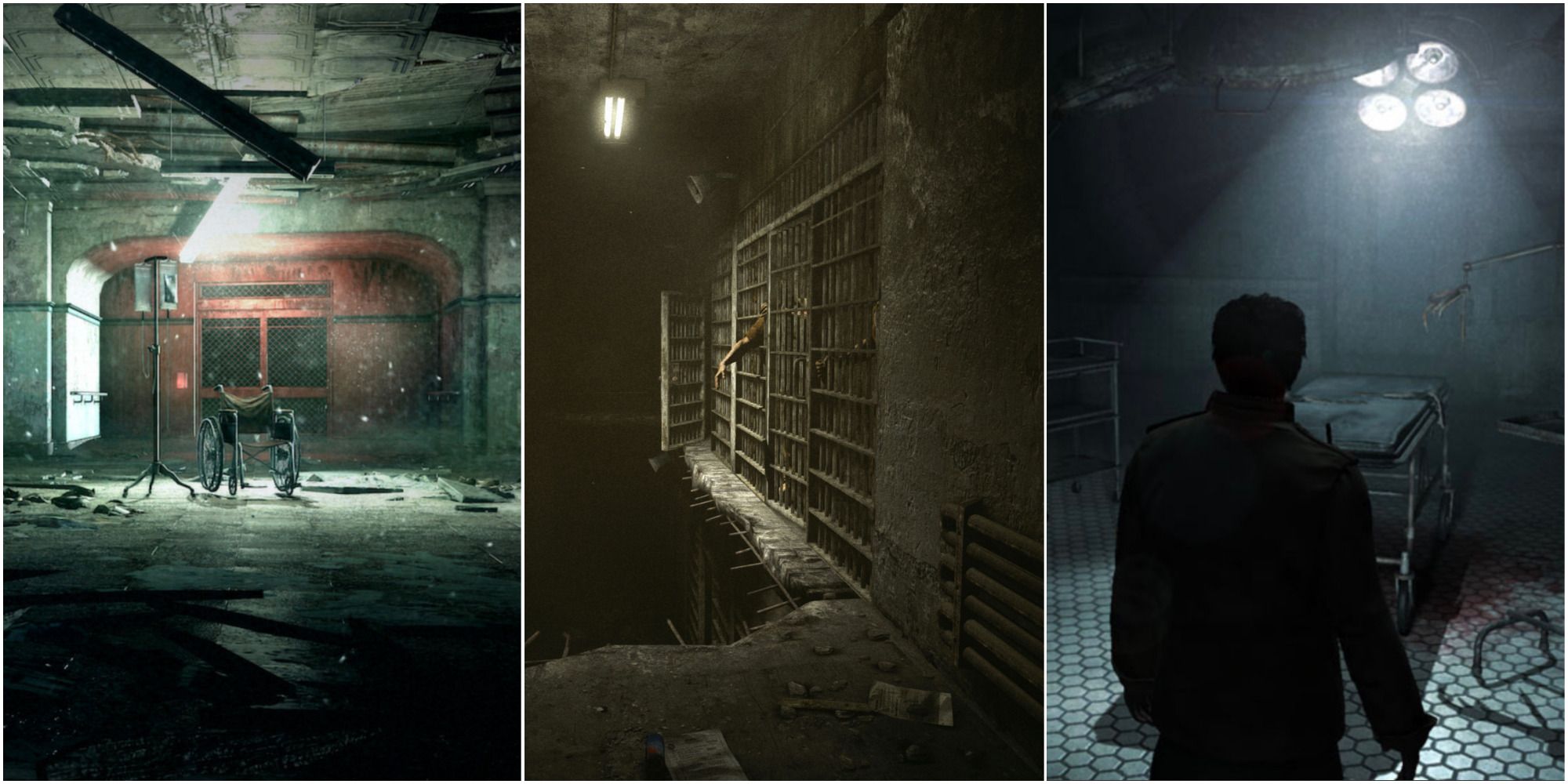Three haunting images are displayed side-by-side, each portraying a dark, evocative scene that feels like a setting from a video game or a horror movie. 

The first image on the left captures a dimly lit, abandoned hospital room. Light filters in from above, illuminating a dilapidated space where ceiling tiles have fallen, and broken fluorescent lights dangle precariously. In the middle of the room stands an old IV pole next to an empty wheelchair, casting eerie shadows. The floor, likely once tiled, is now a grim mix of gray and greenish hues.

The central image is even darker and more sinister, depicting what appears to be a jail cell. Shadows dominate the scene, with a single, faint light source above casting slight illumination. A skeletal arm emerges from behind the grated bars, clutching them as if in desperation. Below the barred door, the floor has collapsed into an abyss, with exposed rebar precariously jutting out, adding to the sense of desolation.

The final image on the right reveals the back of a person wearing a coat, standing in front of an empty, blood-splattered hospital bed in a room with white hexagonal floor tiles. Light shines down upon the floor, creating a stark contrast against the ominous stains, completing a chilling tableau of abandonment and decay.